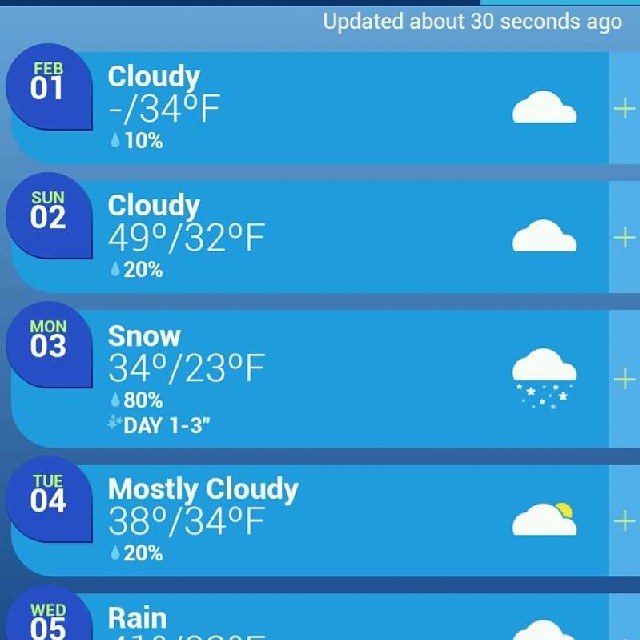The image is a detailed screenshot of a weather report, likely taken from a mobile device. The primary colors are various shades of blue and white, delivering a clean, digital aesthetic typical of weather apps. At the top right, white text indicates the data was "updated about 30 seconds ago." The forecast spans from February 1st to February 5th, with each day listed on the left side inside dark blue, water droplet-shaped backgrounds, and corresponding weather icons on the right.

For February 1st, it shows a cloud icon with a high of 34°F, a low of -34°F being an error, and a 10% chance of precipitation. The February 2nd forecast displays another cloudy icon with a high of 49°F, a low of 32°F, and a 20% chance of precipitation. February 3rd has a cloud with snow falling and predicts a high of 34°F, a low of 23°F, and an 80% chance of precipitation, marking the first day of potential snow accumulation of around three inches. On February 4th, a mostly cloudy icon with some sun is shown, forecasting a high of 30°F and a low of 34°F (likely another error), with a 20% chance of precipitation. The top part of February 5th is visible, indicating rain, although the temperature details are not readable.

The background transitions between darker and lighter blue gradients, organizing the information clearly and visually appealingly. Additional colors noted include green and yellow, possibly highlighting specific data or errors, but are not predominant. The entire image is a single weather app screenshot, with no other objects or backgrounds visible.